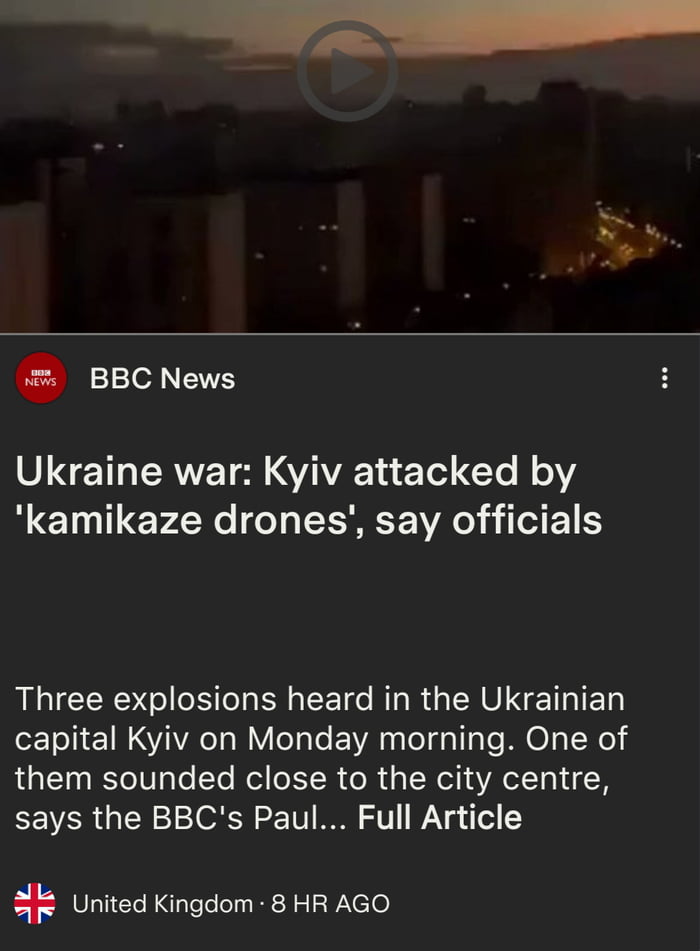The image presents a striking visual against a black background. At the top, there's a dimly lit photograph capturing a bustling city street shrouded in darkness, abundant with traffic. Superimposed on the image is a circle with a right arrow, giving the impression of a play button typically found in video content. 

Below the visual, a horizontal line separates the imagery from the narrative text. The line leads to a red circle with the word "news" boldly inscribed within it. Beside this emblem, the words "BBC News" appear prominently in white font, followed by three ellipsis dots.

The headline reads: "Ukraine war: Kiev attacked by kamikaze drones, say officials." The detailed subtext informs that three explosions were heard in the Ukrainian capital, Kiev, on Monday morning, one of which sounded near the city center, according to the BBC's correspondent, Paul.

Towards the bottom of the text layout, there's a prompt to read the "full article." Additionally, a circle featuring the British flag is situated nearby, accompanied by the note "United Kingdom—8 hours ago," indicating the report's origin and timeliness. All text elements are rendered in a clear, white print for high contrast against the dark background.